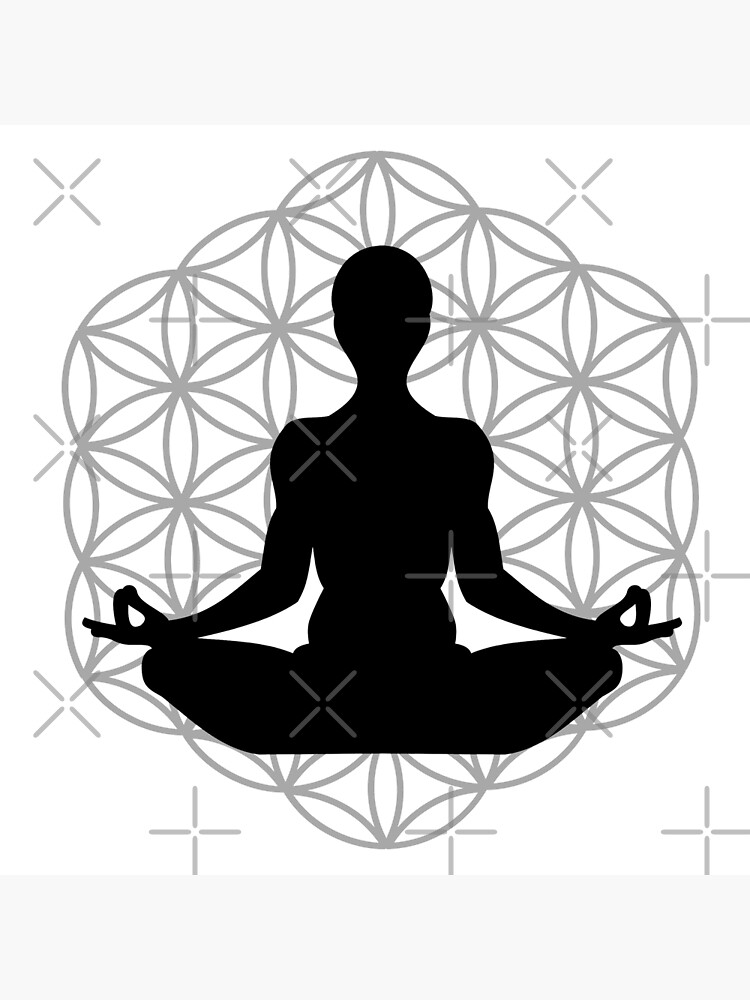The image features a black silhouette of a person seated in the lotus position, commonly associated with yoga and meditation. The individual sits cross-legged with their hands resting on their knees, palms up, and middle fingers touching their thumbs in a gesture of relaxation. The silhouette is stark against a solid white background, emphasizing the figure's front profile. Superimposed on the black silhouette are light gray crosses, Xs, circles, ellipses, and semicircles, forming a complex pattern that engulfs the figure. The entire composition, devoid of any text, is clearly digitally created, with its monochromatic palette restricted to black, white, and shades of gray.